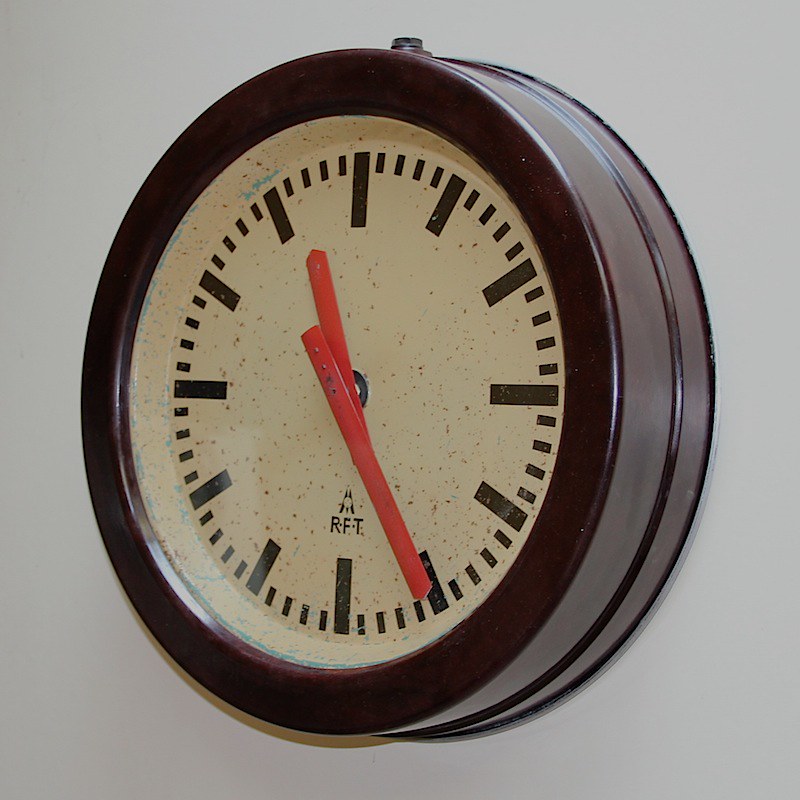This photograph showcases a slightly tilted, circular wall clock mounted on a light-colored wall. The clock seems to be crafted from what appears to be wood with a brown finish, lending it an industrial appearance. The face of the clock is protected by a round glass cover and is bordered by a shiny, silver-colored metal that adds a touch of sleekness. The clock's interior is an off-white or beige color with brown specks, and there is a distinct black frame outlining the face, which gives the clock several inches of depth.

Instead of traditional numerals, the clock features bold, longer black slashes to mark the hours and smaller slashes to distinguish the minutes. The hands of the clock, which display the time as 5:25, are a striking reddish-orange color. Notably, there are blue letters indicating "RFT" positioned approximately where the number 11 would be, and some kind of small symbol just below the hands, adding to its unique industrial charm. The clock carries a sophisticated yet aged look, possibly enhanced by some marks that suggest wear or rust on its surface.